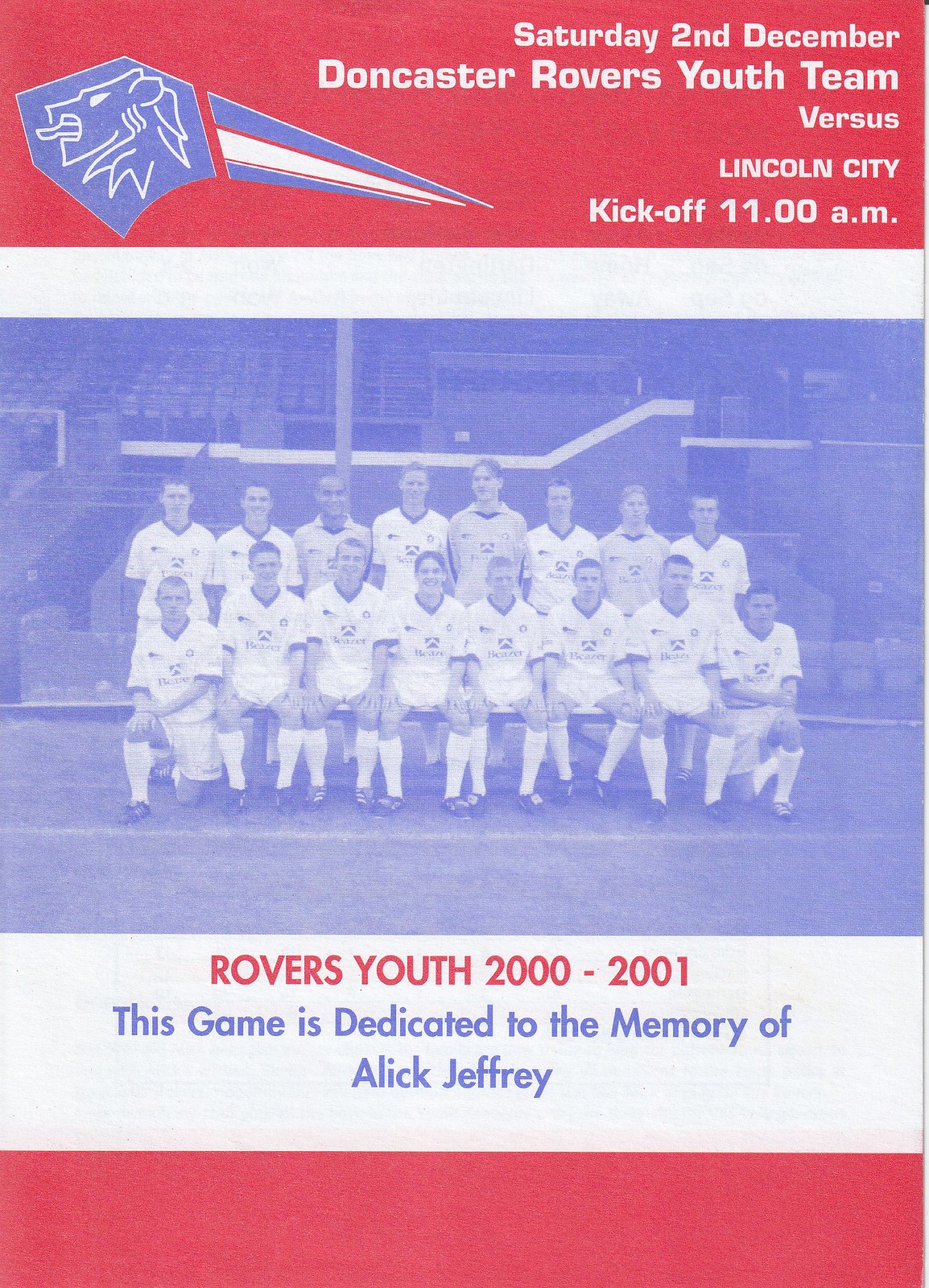This image is a program for the Doncaster Rovers Youth Team, designed in a patriotic palette of red, white, and blue. The top and bottom of the program are bordered in red, with a central white section that includes a striking blue-tinted photograph. The photograph, faded and grainy, features the majority Caucasian youth team dressed in bright white uniforms, with the players arranged in rows—some standing, others kneeling, and a front row sitting. Prominently positioned at the top, in white lettering against the red background, are the event details: "Saturday, 2 December, Doncaster Rovers Youth Team versus Lincoln City, kickoff 11 a.m." An emblem on the left side of the top section depicts a white lion in a blue shape with radiating blue and white lines, presumably the team’s logo. Beneath the team photo, also in red and blue text, are the words "Rovers Youth 2000 to 2001," followed by "This game is dedicated to the memory of Alec Jeffery." The image concludes with another red border at the bottom, completing the patriotic design.